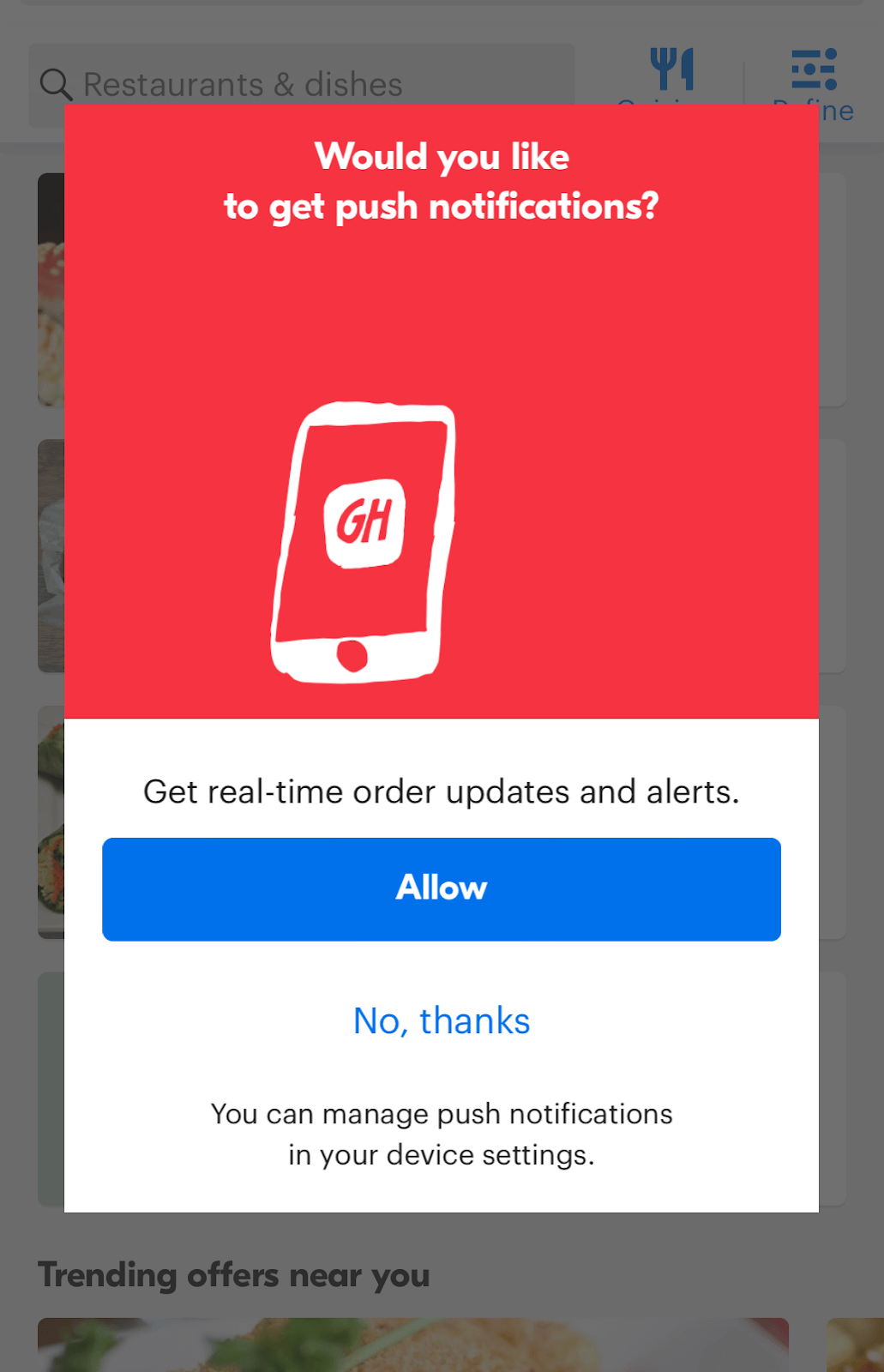The image is a smartphone screenshot, predominantly featuring a prompt asking if the user would like to enable push notifications. The screen is divided into two sections: the top half is red, and the bottom half is white. At the very top in the red section, white text reads, "Would you like to get push notifications?" Below this, an illustrative image of a smartphone is shown, albeit as a very rough drawing. The screen of this sketched smartphone is red with a white center containing the text "GH" and a visible home button. Black text underneath this drawing states, "Get real-time order updates and alerts."

In the lower white portion of the main screen, there are two clickable options. A prominent blue button with white text reads "Allow," and beside it, a link in blue text says "No, thanks." Further below, black text informs the user, "You can manage push notifications in your device settings." Additionally, at the very bottom of the main screen, there is black text stating, "Trending offers near you," along with an icon of a fork and knife, indicating a section related to dining options. The only other visible element is a prominent search bar at the top for restaurants and dishes.